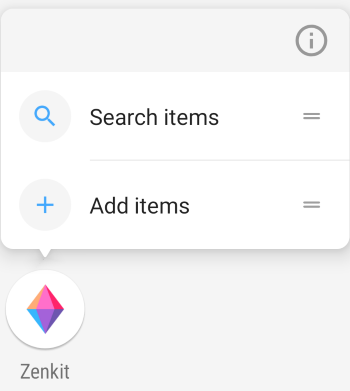A detailed caption for the described image could be:

"The image showcases the interface of the ZenKit app on a device. The screen displays a clean, white background with two primary functional options: 'Search Items' and 'Add Items.' Above these options, in the top right corner, is an information icon represented by a gray 'i' enclosed within a gray circle. The icons for 'Search Items' and 'Add Items' stand out in blue, with the search icon depicted as a magnifying glass and the add icon featuring a plus sign. Additionally, there are two bars on the side, presumably for more options related to the ZenKit app. The app's logo is also visible, consisting of a circle containing a diamond. The diamond is designed to have a 3D effect, with vibrant colors transitioning from top left to bottom right: orange at the top left, red at the top right, pink in the center, blue at the bottom left, purple in the bottom middle, and dark navy blue at the bottom right."